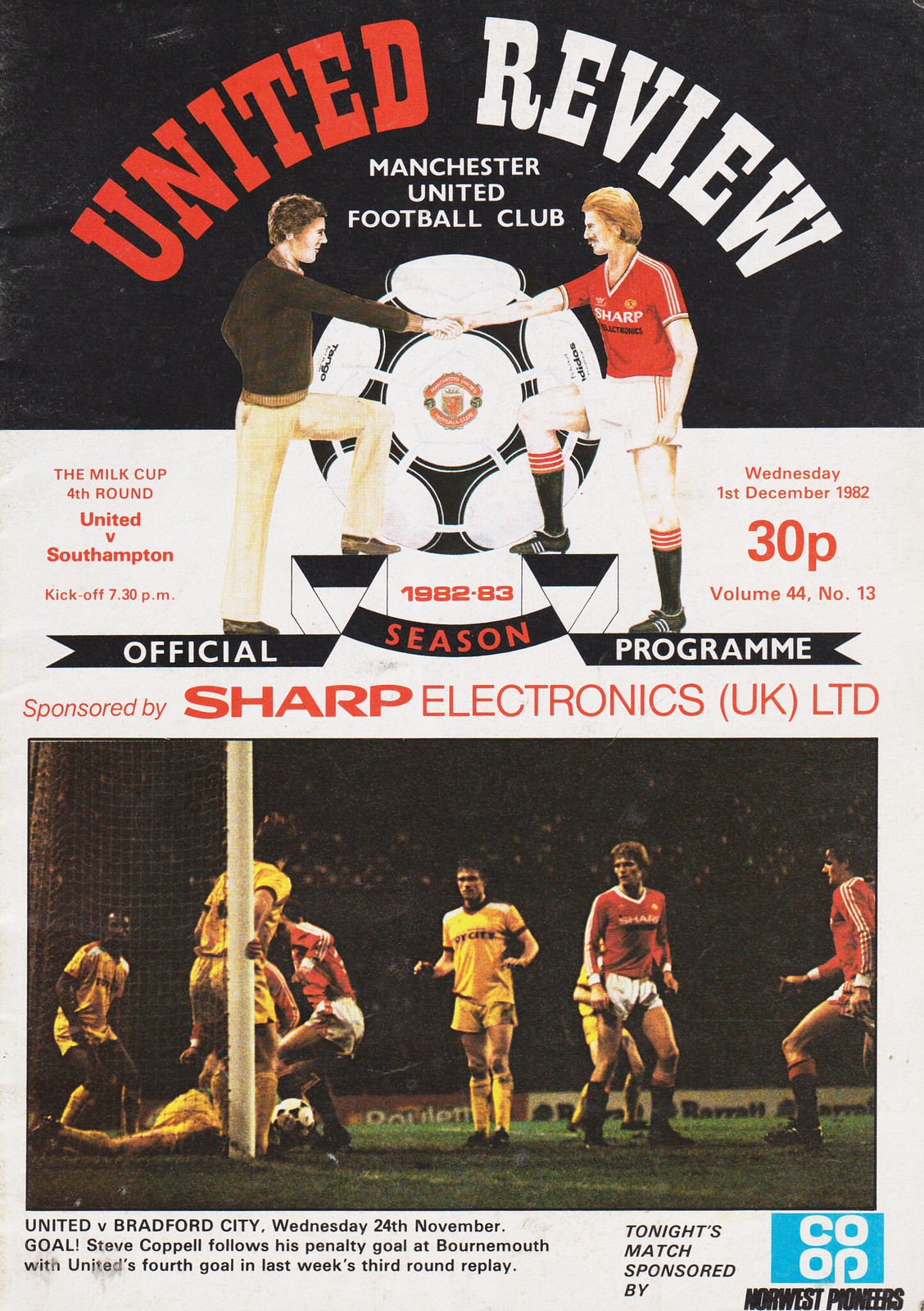This is a page from a vintage magazine, specifically an official Manchester United Football Club program from the 1982-83 season. The program, titled "United Review," features a cover illustration of two men shaking hands. The man on the right is dressed in a red jersey, white shorts, and black socks, while the man on the left wears a brown sweater and white pants. They stand on a cartoon podium with a football behind them, and the 1982-83 season labeling below. The program details the Milk Cup fourth round match between United and Southampton, scheduled for Wednesday, December 1st, 1982, with a kickoff at 7:30 p.m. This volume, number 44, issue 13, was sold for 30 pence and sponsored by Sharp Electronics UK Limited.

Below the main image is a photograph showing a soccer match on a grassy field with teams in red and yellow jerseys. The accompanying text highlights action from a previous game, stating: "United vs. Bradford City, Wednesday, 24th November. Goal: Steve Koppel follows his penalty goal at Bournemouth with United's fourth goal in last week's third round replay." The bottom photograph captures a moment from this night match, which was part of the Milk Cup's third-round replay.